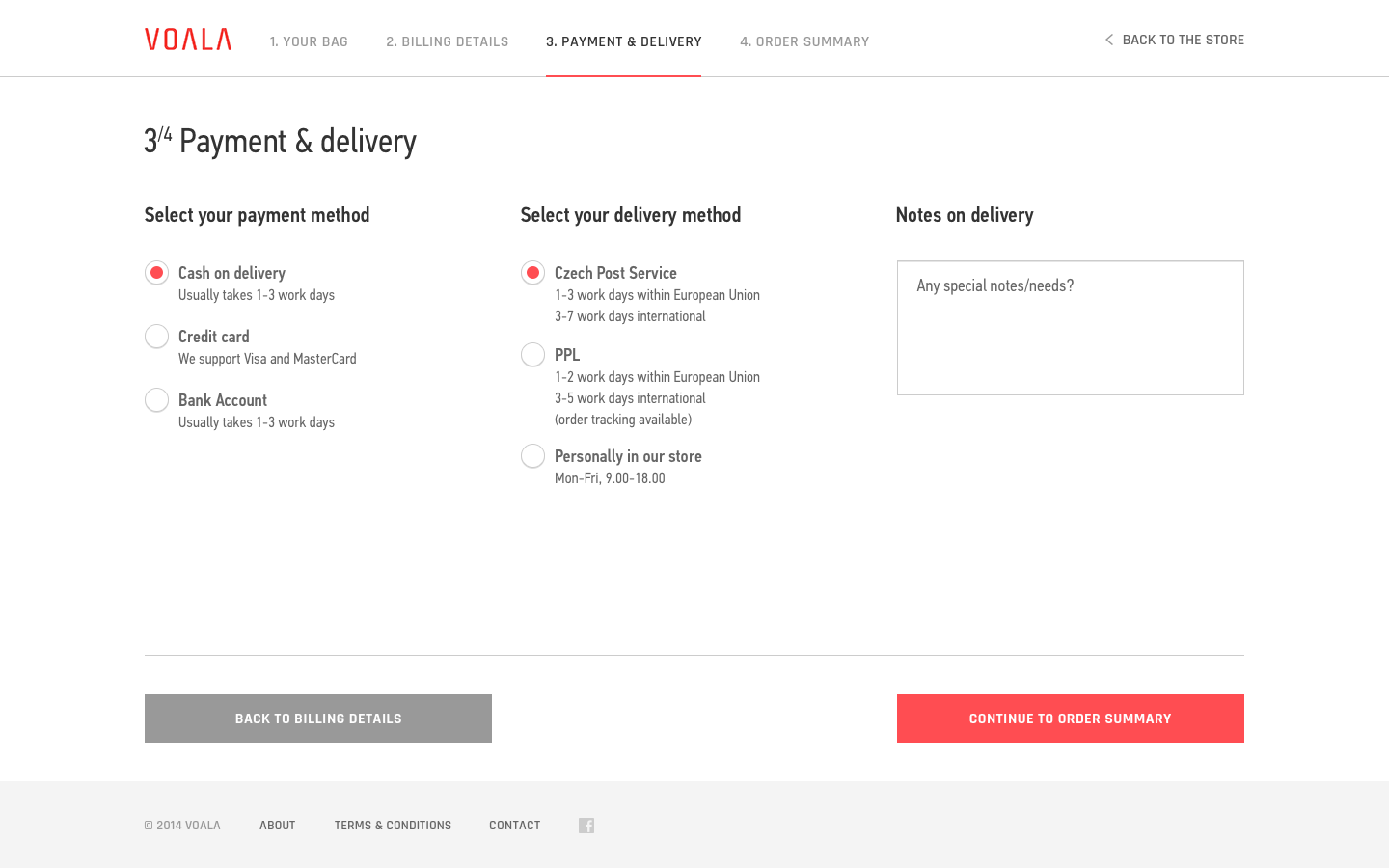The website image for VOALA, spelled V-O-A-L-A, displays detailed data pertaining to a transaction's payment and delivery process divided into three informative columns. The first column, titled "Select Your Payment Method," presents three options: "Cash on Delivery," "Credit Card," and "Bank Account." The "Cash on Delivery" option is currently selected, indicated by a prominent red button. 

In the central column, which is labeled "Select Your Delivery Method," three delivery choices are offered: "Check Post Service," "PPL," and "Personally in Our Store."

The third column, named "Notes on Delivery," includes a text area for entering specific instructions or special requirements related to the delivery, accompanied by an example prompt suggesting the type of notes to be added.

Below the first column is a grayed-out button labeled "Back to Billing Details," while on the opposite side of the screen, there is a contrasting red rectangular button with white text that reads "Continue to Order Summary."